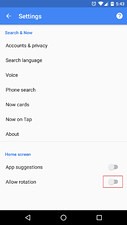This is a screenshot of a smartphone settings menu captured in a vertical rectangular layout. The topmost part of the screen features a thin dark blue border. Below this is a slightly larger border in a lighter shade of blue, containing the word "Settings" in white text aligned to the left, accompanied by a left-facing arrow icon. On the right side of this border lies a white circle with a question mark in its center.

Directly beneath this header is another thin dark blue border. The majority of the screen is occupied by a white section. At the very bottom, there is a black border featuring three navigation icons: a left-facing triangle on the left, a circle in the center, and a square on the right.

Within the main white section, at the top, are blue letters forming the word "Search" followed by an unclear word starting with "N" such as "News". Below this header, in black text, the following menu options are listed: "Accounts and privacy," "Search language," "Voice," "Phone search," an illegible option, "Now on Tap," and "About." A thin gray line separates this section from another set of options.

In the subsequent section, "Home screen" is written in blue letters, followed by options in black text that read "App suggestions" and "Allow rotation."